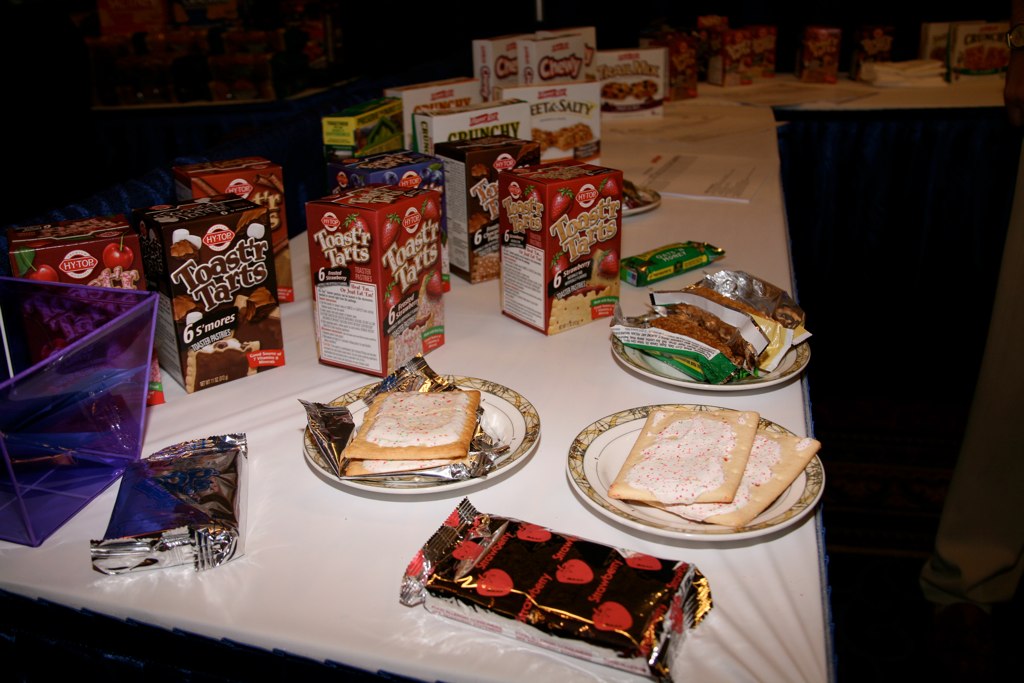This image features an L-shaped arrangement of tables, created by pushing together multiple tables. The photograph is taken from the end of one table, capturing the full span of the L-shape extending to the right. The tables are laden with an assortment of snack packages. Predominantly, these consist of colorful boxes of toaster pastries and granola bars. The packaging includes vibrant hues of red, brown, blue, and white, though the specifics of the text are partially obscured. Visible labels hint at the nature of the contents with words like "Toaster Tarts," "crunchy," "salty," and "chewy." The scene repeats in the background, featuring additional boxes of toaster pastries and various snacks, creating a sense of abundance and variety.